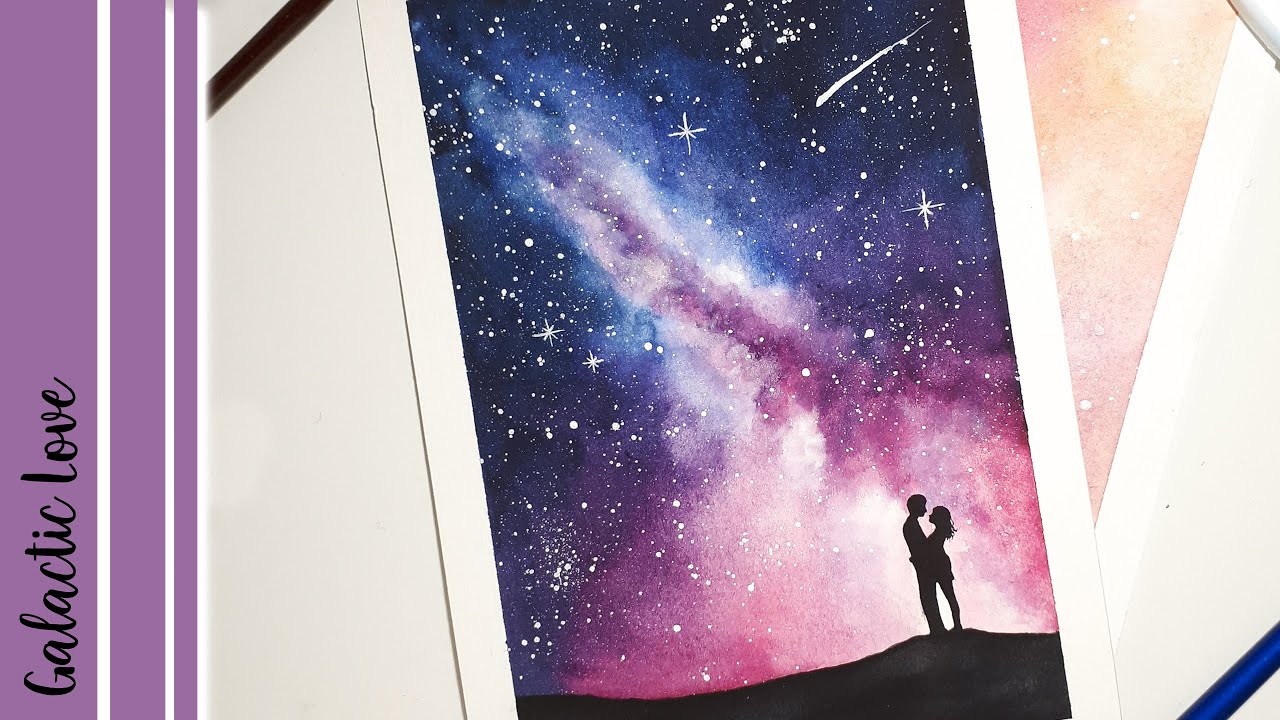The image depicts a romantic artwork centered on a white canvas, showcasing the silhouette of a man and a woman embracing on a dark hill, set against a detailed galaxy-themed background. The galaxy scene features a starry sky with dark blues, bright white stars, a crossing meteor, and a purple gaseous cloud. The silhouetted couple stands in the bottom right corner, looking into each other's faces, evoking a sense of intimacy.

Surrounding the artwork is a structured border consisting of alternating purple and white stripes along the left edge. The first purple strip transitions to a white stripe, then another, slightly narrower purple strip, followed by another white stripe, and finally a third purple strip, all bordered on the far left with the text "Galactic Love" in black print.

The entire scene suggests that the central canvas is placed on a white table, with glimpses of another piece of paper partially covered underneath. Three pencils—a blue, a white, and a brown—lie on the table, which might be decorative elements. The setting feels like a digital composition depicting a series of artworks layered together, giving the impression of an artist's workspace.